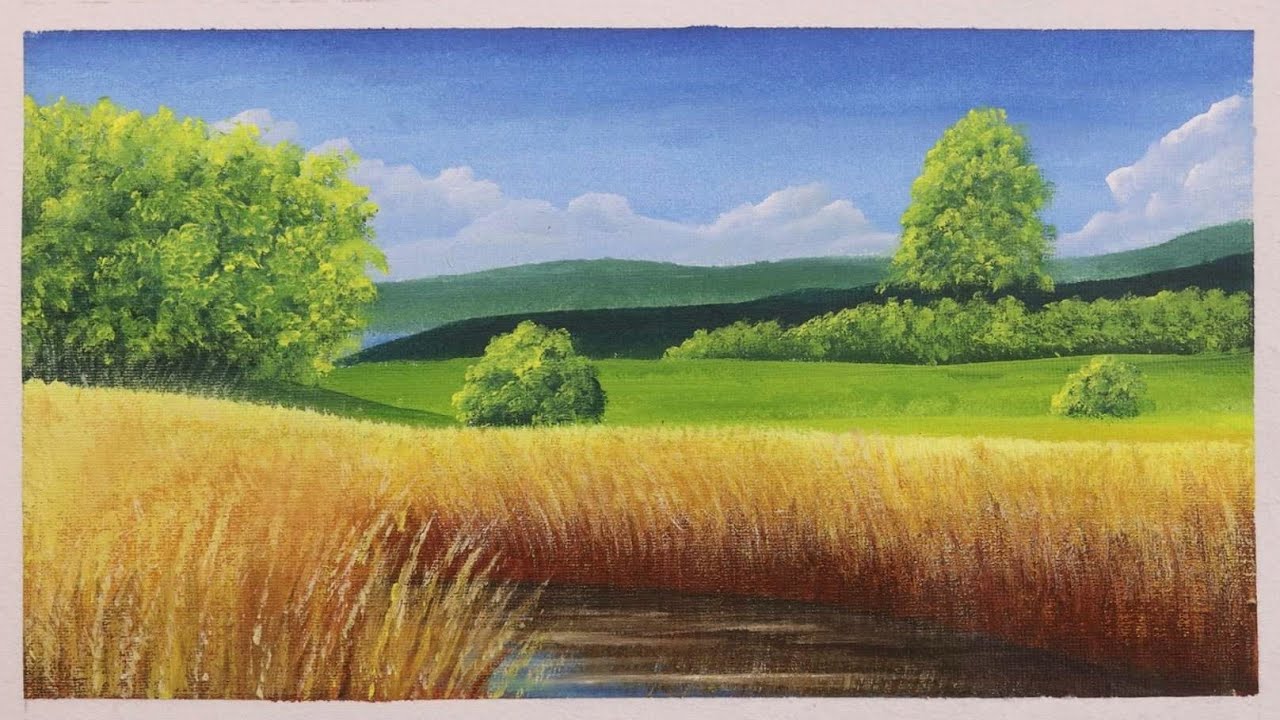This serene horizontal painting beautifully captures the essence of a natural area, presenting the viewer with a peaceful landscape. At the top of the painting, a bright blue sky transitions into various shades of blue, adorned with large, fluffy white clouds. The background reveals rolling hills, some faintly green-gray and others a darker, charcoal shade, creating a sense of depth. A mix of greenery features prominently throughout; on the left side, there's a large bush with a smaller one beside it, while to the right, a clump of dark green bushes stands tall. In the middle ground, a bright green grassy field stretches out. The foreground, which draws the viewer's eye, is dominated by tall golden and orange grasses, their tips ranging from tan to gold to ivory. The grasses partially obscure a waterway that reflects the scene, giving a hint of a peaceful, reflective surface. The overall effect is a tranquil, cohesive scene that evokes a sense of calm and natural beauty, suggesting the possible use of oil paints to achieve the vibrant colors and textures.